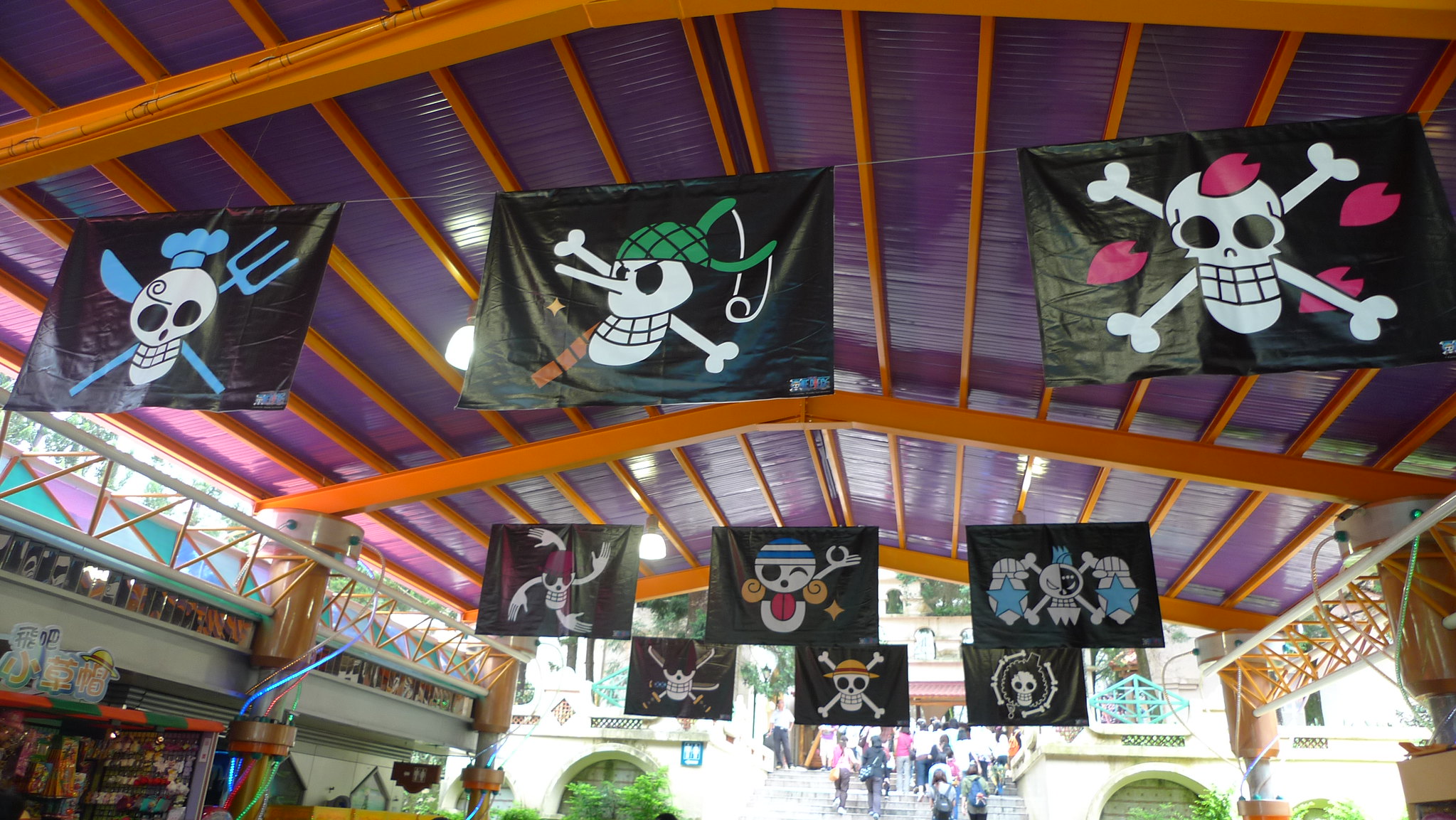This photograph captures an intricately designed ceiling of what seems to be an outdoor gift shop or store, adorned with animated, cartoonish flags suspended from white cords. The ceiling features a striking mix of light purplish and pinkish hues embedded in a silvery metallic surface, complemented by dark yellow-orange wooden support beams. Hanging from the ceiling, there are nine prominently displayed flags, each set against a black background and featuring various stylized skull and crossbone designs. Notably, these include recognizable elements from popular anime, such as one flag resembling the One Piece emblem with a skull wearing a straw hat. Other flags showcase unique details: one has a blue chef's hat alongside a fork and knife, another is embellished with pink hearts, and yet another features what looks like a green hat. In the background, additional similar flags can be seen extending into the distance, further enhancing the whimsical atmosphere. Below, a group of children or students are visible, seemingly heading towards a school, adding life to this lively, vibrant scene.